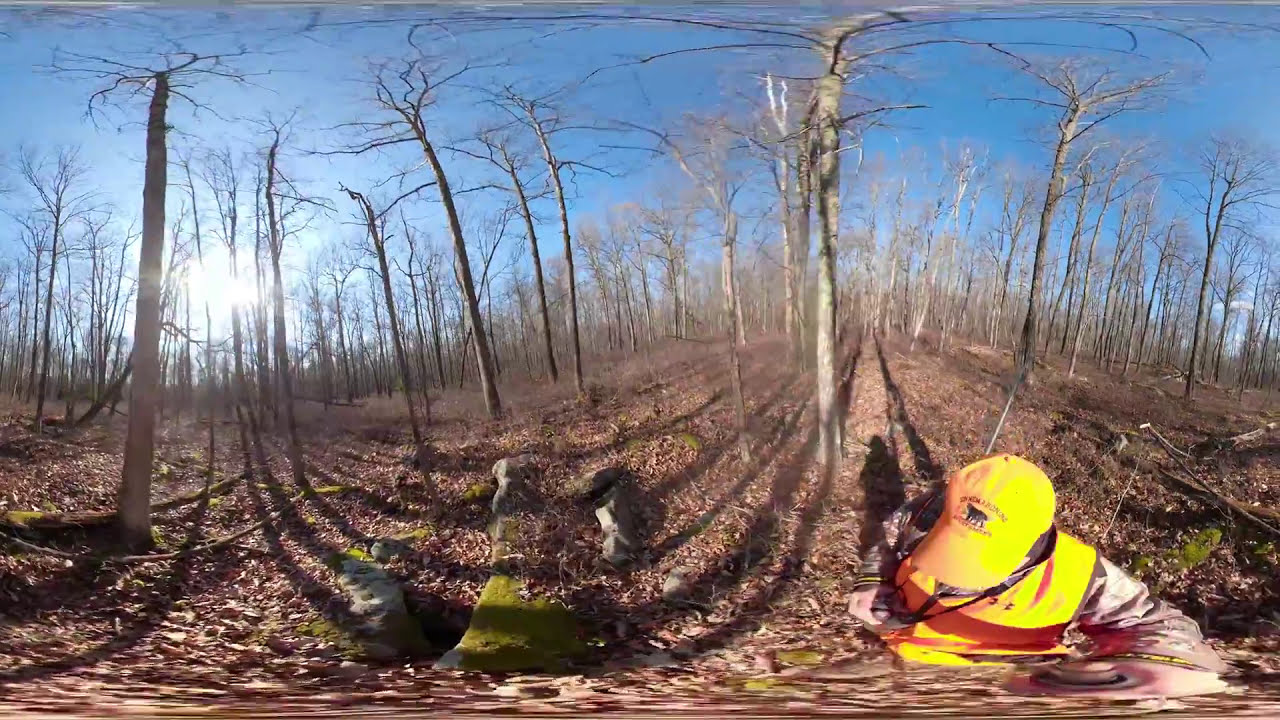This panoramic and highly distorted image captures a desolate forest scene, likely during late autumn or early winter. The forest is filled with tall, leafless trees stretching out their long, gray branches against a clear, bright blue sky. The sun, positioned in the middle left of the image, shines strongly, casting a stark light across the landscape. The ground is blanketed in a thick layer of brown and reddish dead leaves, contributing to the desolate atmosphere. In the bottom right of the image, a person is partially visible, wearing a bright yellow-orange baseball hat featuring a logo of a quadruped and some black text, along with a matching vest. They also sport a gray or tan long-sleeve shirt. Moss-covered rocks are scattered throughout the forest floor, adding a vibrant green contrast to the otherwise muted palette. The distorted proportions due to the 360-degree camera perspective add an unusual curvature to the scene, further enhancing the eerie, otherworldly feel of the image.